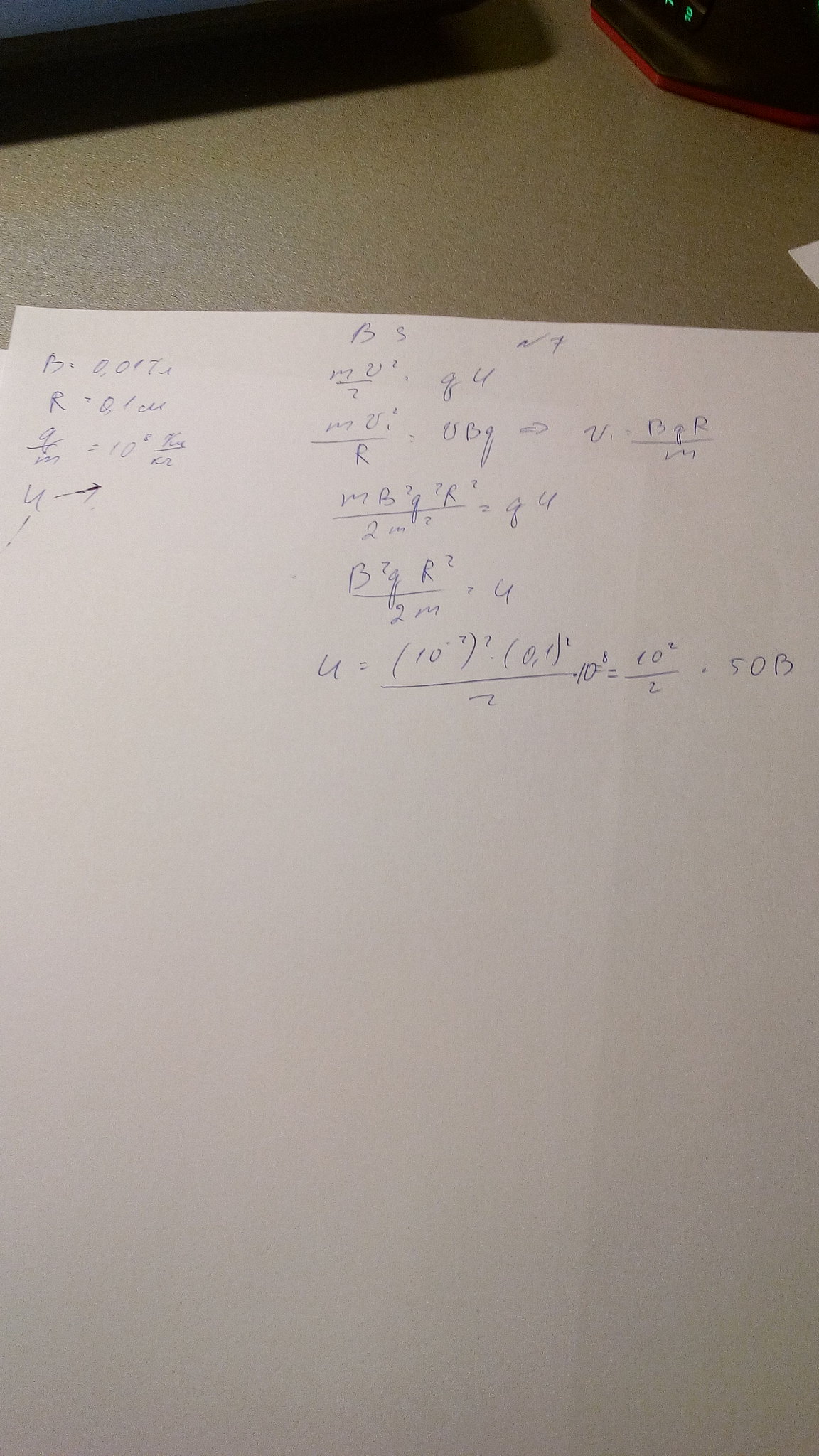The image depicts a white sheet of paper populated with numerous handwritten mathematical equations in blue pen. The equations are intricate and clutter the page, making them somewhat challenging to decipher. 

**Detailed Breakdown of the Equations:**
1. The foremost equation on the left begins with "B.00T" followed by "R.QT" and continues as "QM x 10 KM / ? CM."
2. Below this equation, another sequence includes characters such as "U," an arrow, and an exclamation mark.
3. In the top-right corner of the paper, "BS/7" is written. Directly underneath, it says "MU2 / 2 * QU," followed by "MU2 / R.UBY arrow U.BQR / M."
4. Another complex equation states, "MB2Q2R2 / 2M2 = QU."
5. Further down, the equations "B7Q R2 / 2M.U" and "U = (10^-7) (7. (0.1) 2 / 2 * 10^2 = 10^2 / 2 * SOB" are also present.

**Context and Surroundings**:
The paper rests on a beige countertop. In the background, there's a black machine with a red base. The top-left corner of the image shows another black object, and above the paper is another white item.

Overall, the image captures a complex set of mathematical equations scribbled hurriedly on a white sheet, framed by a beige countertop and miscellaneous objects in the background.